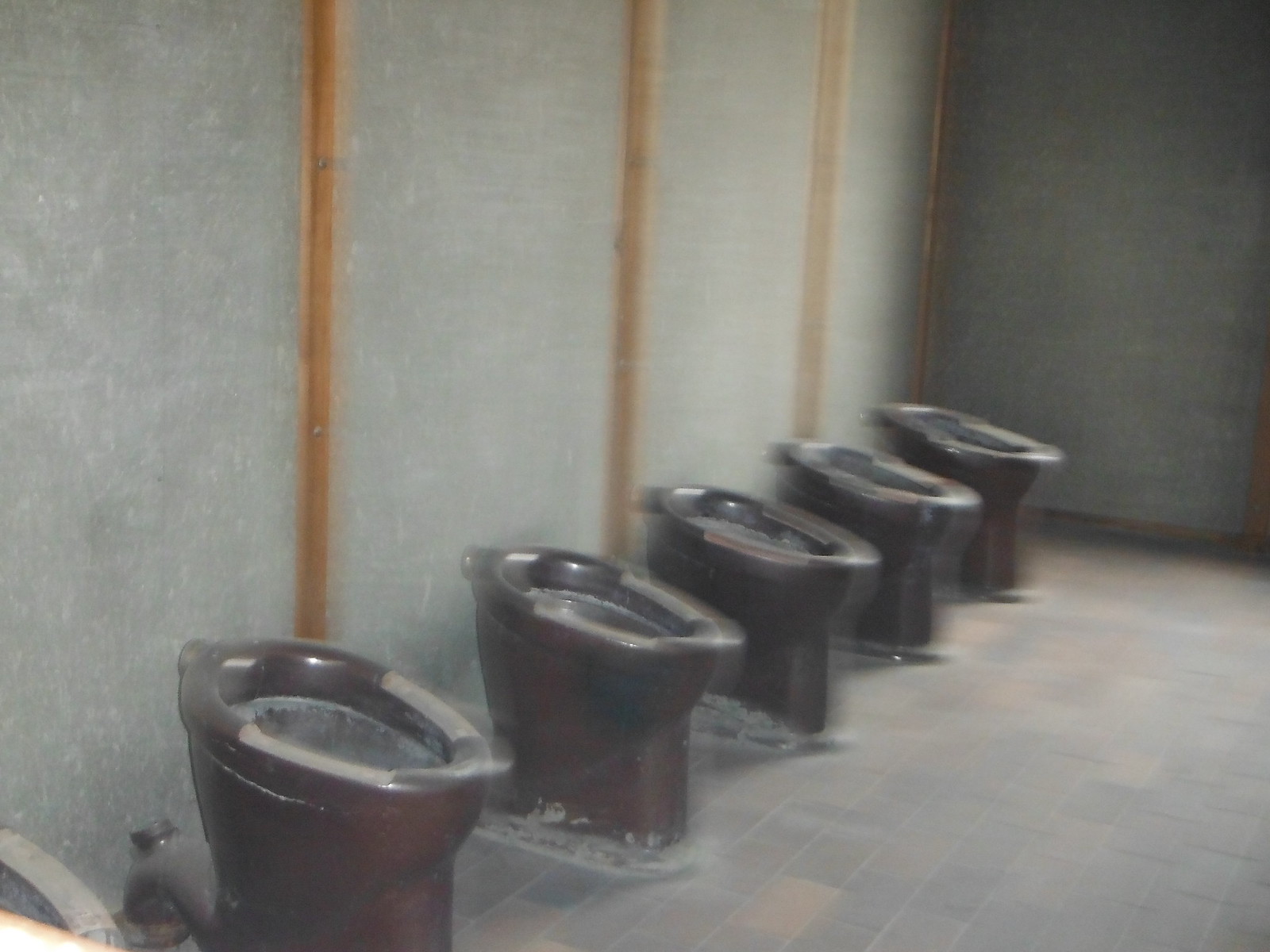This image depicts a somewhat blurry view of a room with five black toilets positioned in a linear arrangement along the lower left corner of the space. The bowl of a sixth toilet is partially visible. The toilets lack the upper tanks and instead have light gray pads on the seats with some light gray grime or dirt around the rims of two of them. The walls are a dark gray color, accented with three vertical wooden panels. The floor features a pattern of gray tiles slightly darker than the walls, interspersed with lighter brown or rust-colored tiles, giving it a somewhat dirty and dusty appearance. Despite the image's blur, the overall deteriorated state of the room is evident.